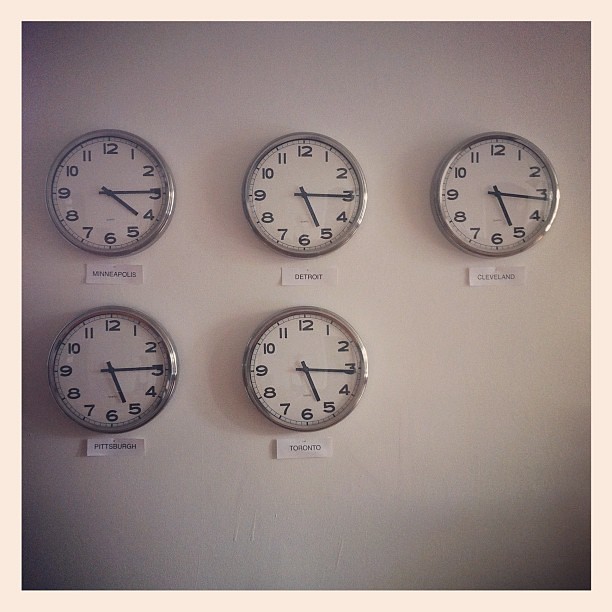In this image, five clocks are mounted on a wall in a somewhat asymmetrical arrangement, consisting of three clocks on the top row and two on the bottom row. The bottom row is aligned perfectly in a column with the top two clocks, but the bottom right corner is conspicuously missing a sixth clock, which disrupts the visual balance and creates a sense of incompleteness.

Each clock features a classic design with a white face, black numerals, and a silver or chrome outer border. The top row displays clocks labeled for Minneapolis (left), Detroit (middle), and Cleveland (right). The times shown are approximately 4:14 for Minneapolis, 5:16 for Detroit, and 5:17 for Cleveland. The bottom row consists of clocks for Pittsburgh (left) and Toronto (right), indicating times of 5:14 and 5:16, respectively.

The irregular arrangement and potentially incorrect times contribute to a visually and functionally unsatisfactory display. Adjusting the placement of the bottom two clocks could improve the overall balance and aesthetic appeal of the display.